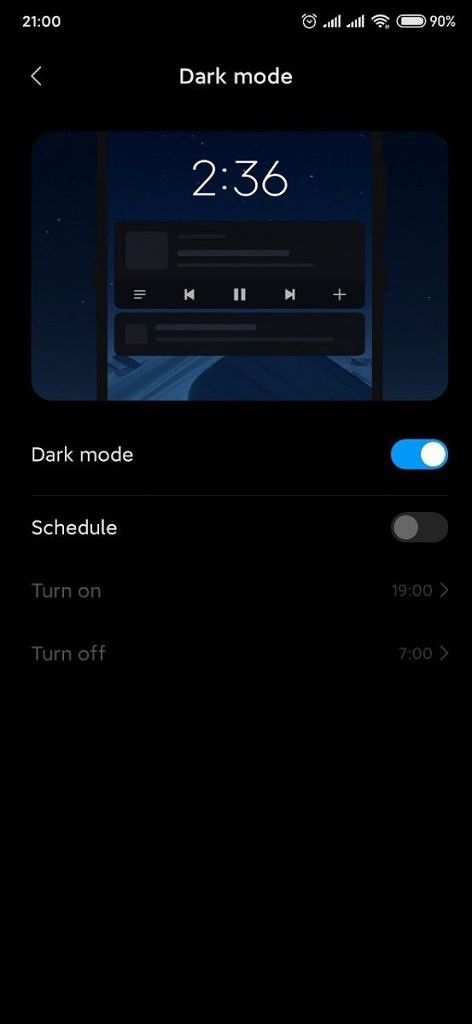The image displays a portrait-oriented screenshot of a cell phone screen with a black background. The top left corner shows the time, "2100" or 9:00 PM, and the top right corner features typical cell phone status icons, including a 90% battery indicator, signal strength bars, and an alarm clock symbol. A left-pointing caret in white is positioned in the top left corner. Centrally, the words "Dark mode" are prominently displayed, consistent with the dark screen theme.

Below this title, there's a graphical representation of a cell phone screen in dark mode, enclosed within a rectangle with rounded corners. The screenshot appears to be a screen capture of the phone's dark mode settings.

Beneath this rectangle, there are toggle switches for adjusting dark mode settings. The "Dark mode" toggle is activated, indicated by a white radio button and a light blue slider. Other options, such as "Schedule," "Turn on," and "Turn off," are present but grayed out, indicating they are not currently selected. The image illustrates a user configuring their cell phone to stay in dark mode, likely for ease of viewing in low-light conditions or personal preference. The specific model of the phone is not identifiable from the screenshot.